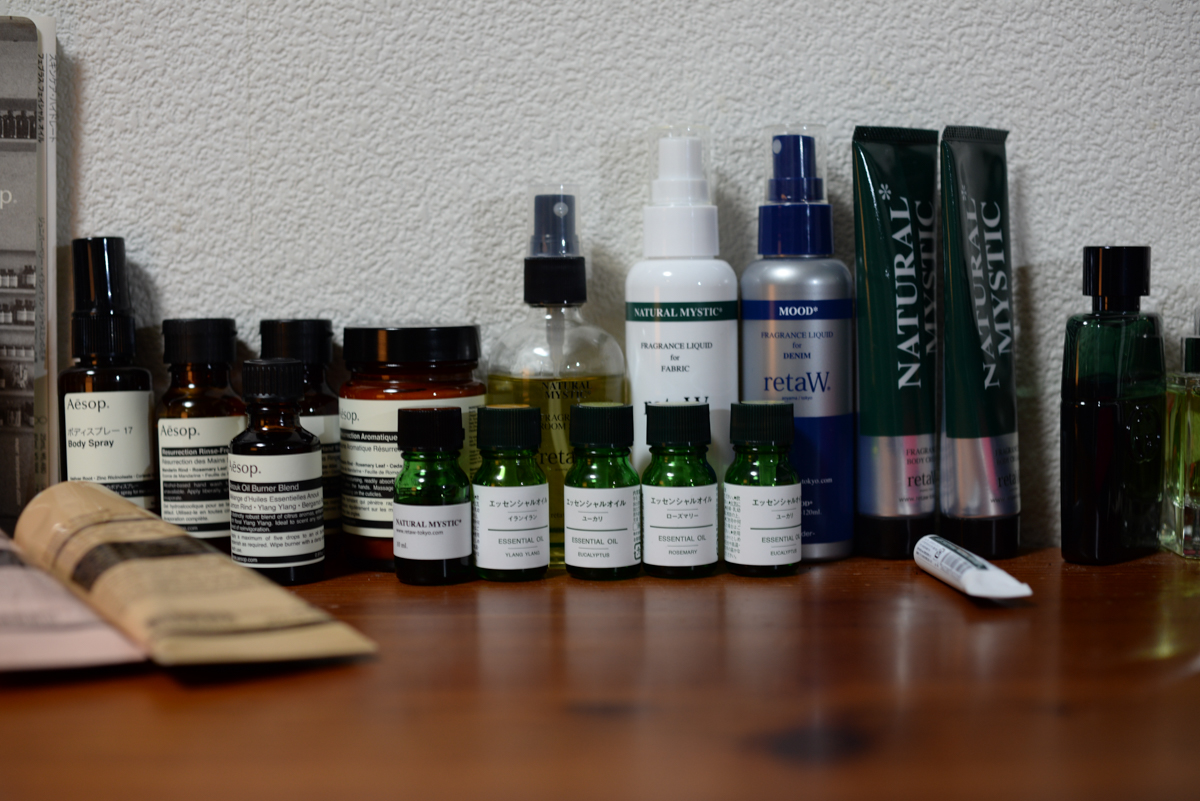This detailed photograph captures an assortment of various bottles and tubes neatly arranged on a wooden table. In the center, a group of approximately twelve small glass bottles is prominently displayed. Among them, some are green, others have a brown hue, and one stands out with its clear glass. Several of these bottles bear the label "Aesop," indicating the brand.

To the right of the cluster of small bottles are two notably larger bottles. The first larger bottle is white, while the second one is dark blue with the word “Mood” clearly printed on its label. Adjacent to these are two dark tubes, primarily black with silver accents at the bottom, and both tubes have partial text visible, including the word "natural." In front of these black tubes, a smaller white tube lays horizontally.

On the far left of the arrangement is another tube, which appears somewhat browned out, also lying flat on its side. The mix of colors and shapes creates a visually interesting and diverse collection of products on the rustic wooden surface.